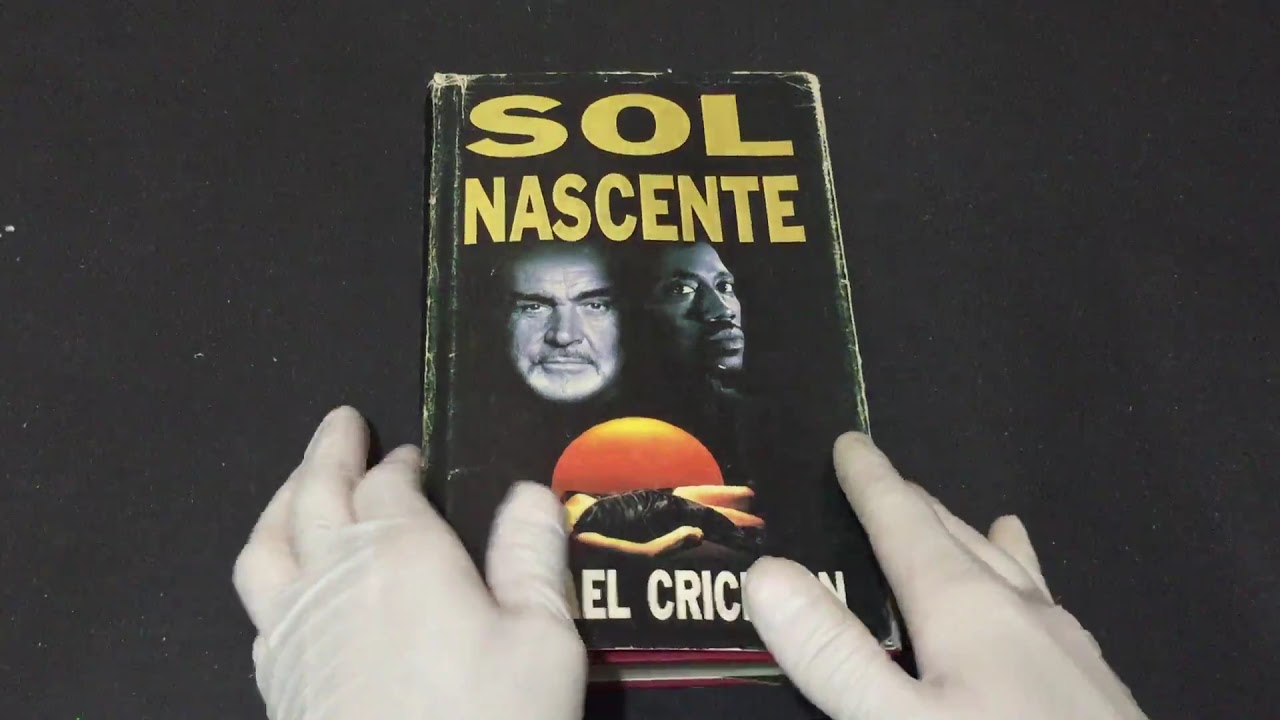This is a detailed photograph of a worn book with a black cover, lying on a black surface. The book's title, "Sol Nascente," is prominently displayed at the top in yellow font. Central to the cover are images of two men, with an older white man and a younger black man. Below them is a depiction of a woman lying on the ground with a large red and yellow sun setting behind her. The bottom part of the cover features the author’s name, partially obscured by a pair of gloved hands—the hands are covered in white gloves, suggesting careful handling. The visible characters on the cover suggest the author's name includes "E-L" and "C-R-I-C-N." The book appears well-used, with wear showing as white marks around the edges and the binding. The photograph captures a sense of age and handling, with minor specks noticeable on the black surface beneath the book.